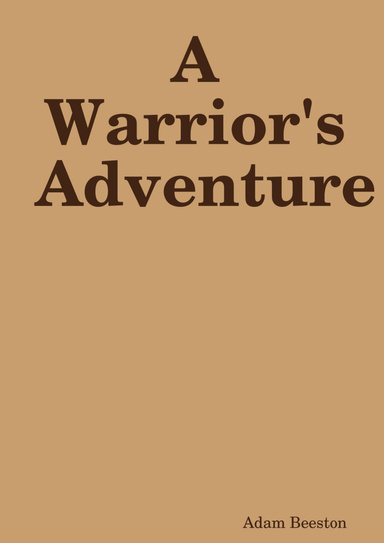The digital image appears to be a proposed book cover featuring a plain, minimalistic design. The background is a solid dark tan color, giving it an understated appearance. Dominating the upper portion of the image, the book's title, "A Warrior's Adventure," is inscribed in large, dark brown text. The title is segmented across three rows, with "A" on the first row, "Warrior's" on the second, and "Adventure" on the third. In the bottom right corner, the author's name, "Adam Beeston," appears in a smaller, similarly dark brown font. The text colors almost approach black, creating a stark contrast with the lighter background. The overall image is notably simplistic, devoid of any additional artwork or intricate detail, suggesting it could have been quickly crafted using digital design software such as Photoshop.